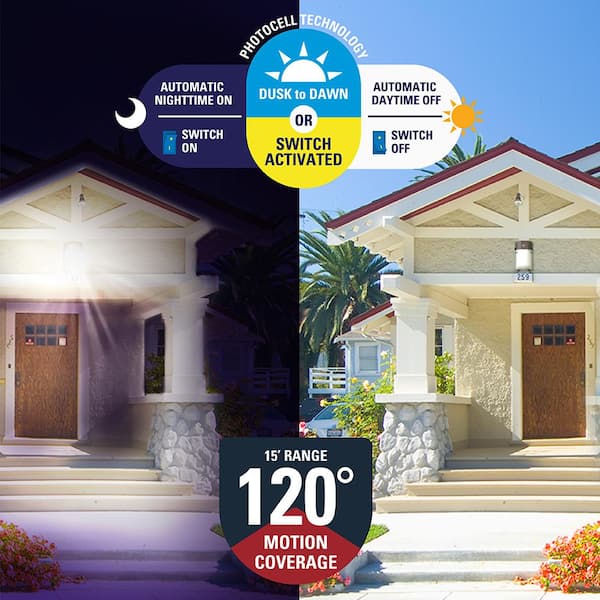This image is an advertisement for a home lighting and security system developed by PhotoCell Technology. It features two side-by-side photos of houses: one taken at night showing an illuminated home, and the other taken during the day with the lights off. 

At the top, the advertisement boasts "PhotoCell Technology," with labels for "Automatic Nighttime On" and "Switch On" on the left side, and "Automatic Daytime Off" with "Switch Off" on the right side, accompanied by icons representing a sun and a switch. The center of the image highlights a "Dusk to Dawn" feature, indicating that the system can be activated either by natural light changes or manually via a switch. 

The advertisement further details the product's specifications at the bottom, noting a 15-foot range and 120-degree motion coverage. An illustration of a bright light with rays emanating from it emphasizes the system's effectiveness in low-light conditions.